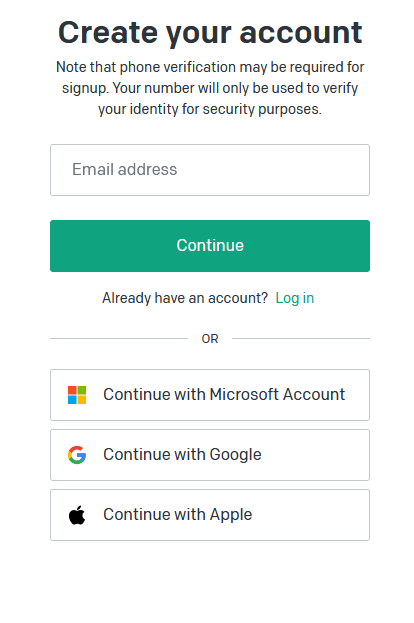At the top of the image, there is a prominent heading that reads "Create Your Account" in large, bold, black letters. Directly below this, in smaller sans-serif black text, there is a note stating, "Note that phone verification may be required for sign up. Your number will only be used to verify your identity for security purposes."

Beneath this informational text is a light gray rectangle containing the placeholder text "Email address" in gray. Below this rectangle is a solid green button of the same size, featuring the word "Continue" in white type.

Further down, there is a sentence that reads, "Already have an account?" with the word "Login" to its right in green text. Separating the sign-up options, there is a horizontal gray bar with the word "or" in the center, flanked by gray bars on either side.

Below this separator, there are three horizontal rectangles providing alternative sign-up methods:
1. The first rectangle displays the Microsoft logo, which consists of four smaller squares in red (top left), blue (bottom left), green (top right), and yellow (bottom right), alongside the text "Continue with Microsoft account."
2. The second rectangle features the Google "G" logo, with its signature red, yellow, green, and blue colors, followed by the text "Continue with Google."
3. The last rectangle includes the black Apple icon with the accompanying text "Continue with Apple."

This image thoroughly guides a user through various account creation options and highlights potential methods to sign in by leveraging existing accounts such as Microsoft, Google, or Apple.